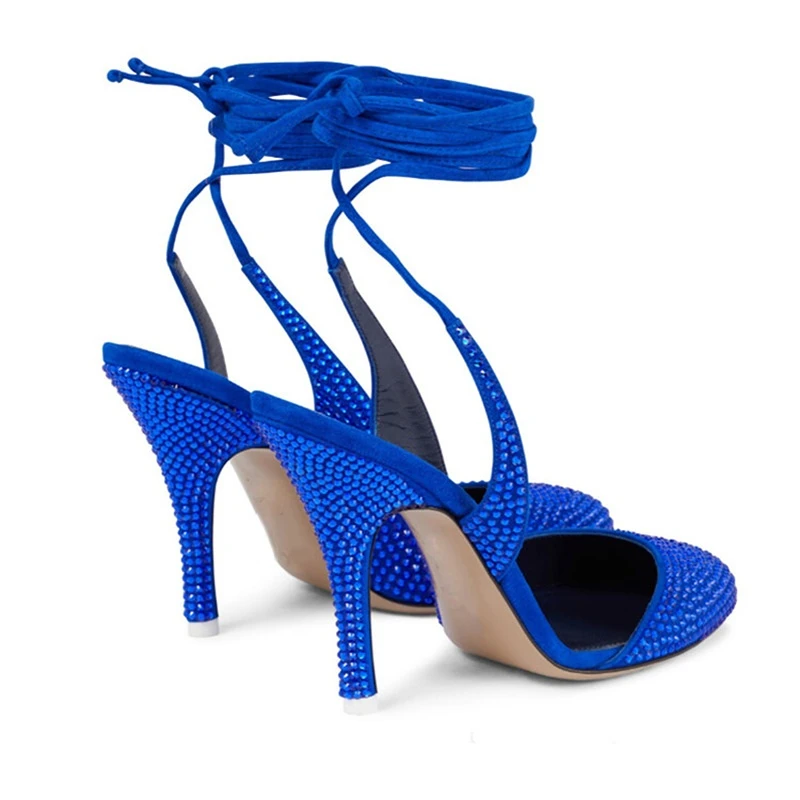This photograph features a pair of high-heeled shoes set against a white background, capturing the essence of a fashion advertisement. The shoes are a striking royal blue with a studded texture resembling small, uniform pinheads or beads, giving them a unique, non-smooth finish. They feature ankle straps that ascend upwards, possibly extending to the calf, and these straps are tied into an elaborate, neatly round shape that appears to be floating above the shoes. The shoes have beige soles and white caps on their approximately 3-inch heels, adding a hint of contrast to the otherwise monochromatic blue design.